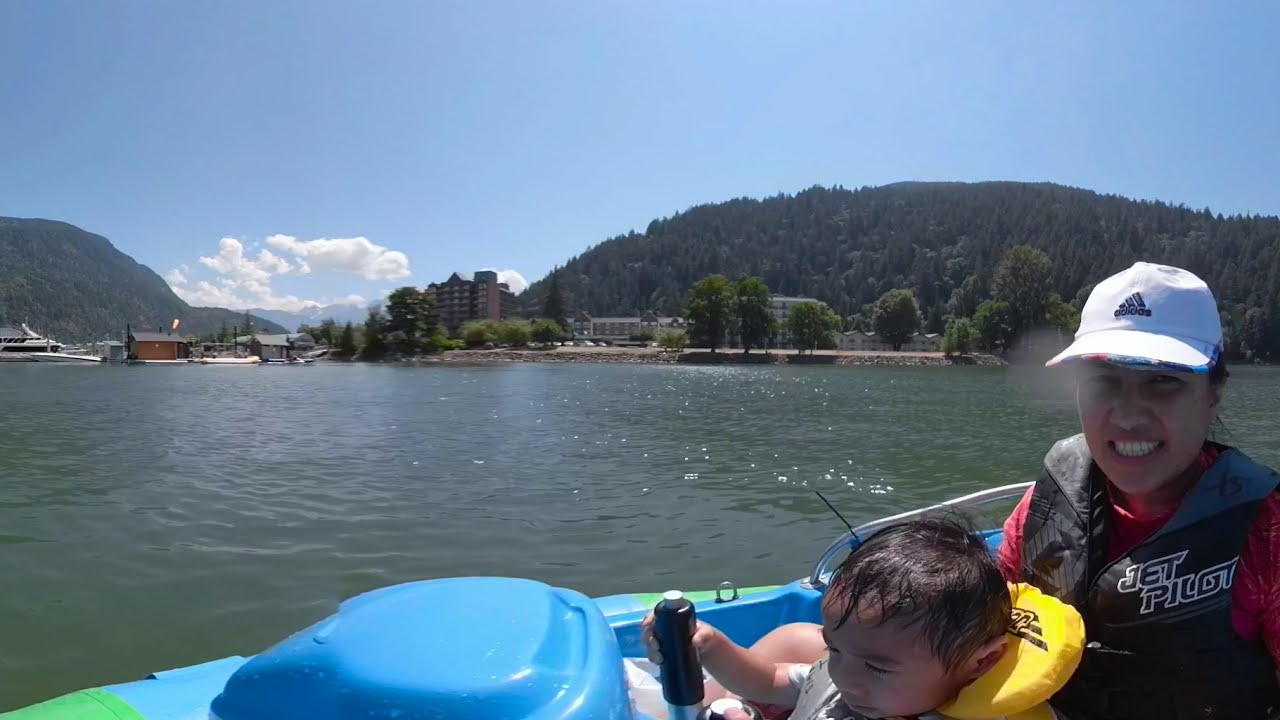In the foreground of this vivid color photograph, a little boy in a yellow life jacket sits on the lap of a woman wearing a black life vest labeled "Jet Pilot" and a white Adidas hat. They are both seated in a blue and green kayak positioned at the bottom left corner of the image. The boy holds a black water bottle while they navigate a dark green body of water that extends to the midpoint of the picture.

Beyond the water, several boats are docked at a harbor in the central part of the image, with a cluster of buildings, including a large cabin or hotel, visible in the mid-background. The right-hand side features more facilities with a utilitarian look. Towering hills densely covered with green trees rise behind these structures, adding a natural backdrop to the scene. Above it all, the sky is a clear light blue, adorned with a few fluffy white clouds, suggesting a beautiful and sunny day.